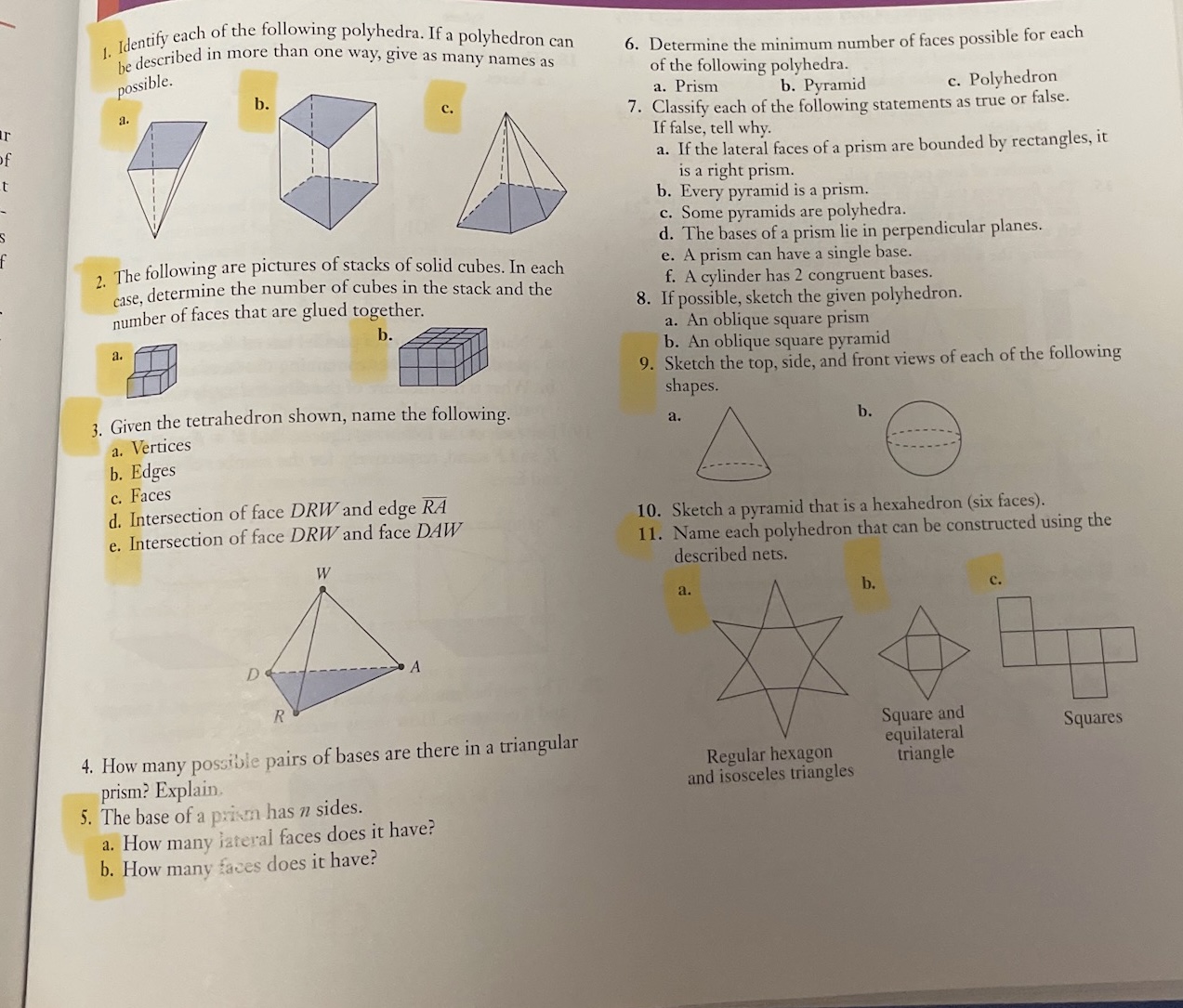This photograph reveals a detailed page from a math textbook, oriented around the study of geometric shapes and polyhedra. The page is divided into two wide columns of text and exercises, with questions numbering from one to eleven. At the top of the left column, there are diagrams of polyhedra marked A, B, and C—A being an upside-down 3D triangle, B a 3D cube, and C another 3D triangle. The first question instructs: "Identify each of the following polyhedra. If a polyhedron can be described in more than one way, give as many names as possible." 

Proceeding to the second column, the geometric theme continues with more complex shapes and questions. The second question requires identifying stacks of solid cubes and determining the number of cubes and faces glued together. Subsequent questions delve deeper into polyhedral properties and recognition. Question three, for example, asks for the identification of vertices, edges, faces, and specific intersections of a labeled tetrahedron. 

The page is rich with further queries that challenge understanding of geometric principles, such as recognizing the pairs of bases in a triangular prism, calculating faces in prisms and pyramids, classifying statements as true or false about prisms and polyhedra, and sketching oblique polyhedra and views of shapes. The text and diagrams throughout are systematically laid out, some highlighted in yellow for emphasis. Notably, additional shapes like a blue ink party hat outline, circular and star outlines, add visual variety to the learning material.